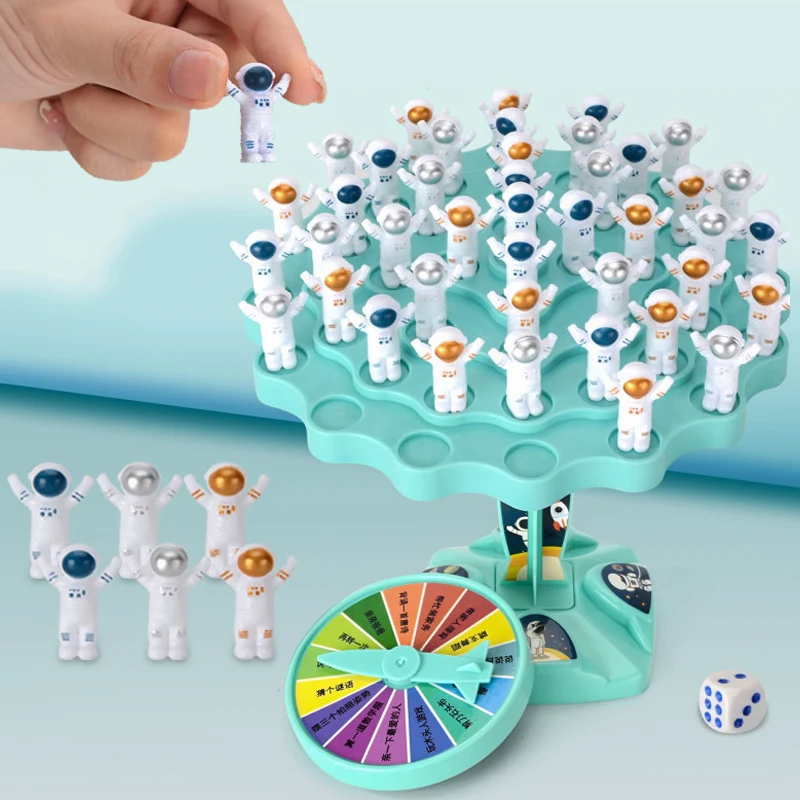The image depicts a children's game centered around a plastic tree-like pedestal with various small, circular holes. The tree, primarily green in color, is adorned with miniature astronaut figures dressed in white suits. These astronauts have visors in different colors—orange, blue, silver, and gold. Most of the slots on the pedestal are occupied by these figures, and one hand is visible, about to place another astronaut into a vacant hole. Additional astronauts, yet to be placed, sit on the surface below, grouped by visor color: two blue, two silver, and two orange. At the base of the pedestal, there's a meter or spinner with an arrow, displaying sections in multiple colors—ranging from red, orange, and brown to various shades of green, yellow, pink, and purple—with text in Chinese or Japanese. A small white die with blue dots showing the numbers two, three, and six lies adjacent to the game setup.